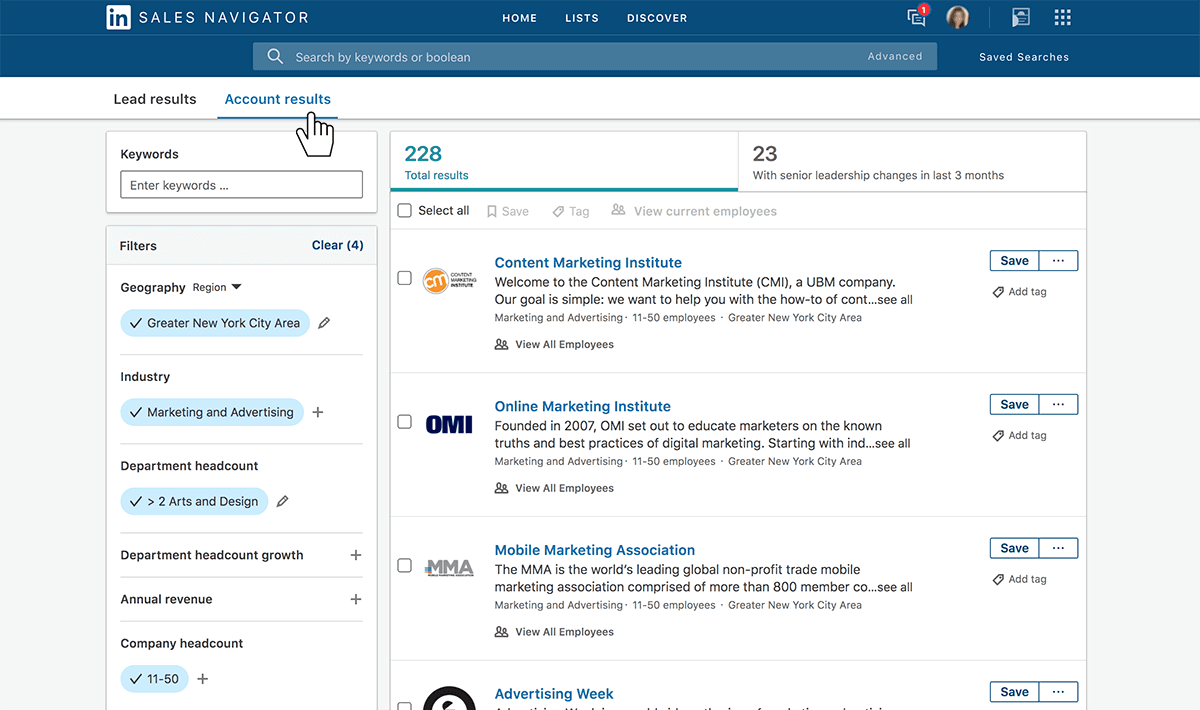"Screenshot of a job search results page showcasing detailed search filters and listings. At the top of the page, a circular avatar displays a woman's photograph. Beneath it, a search bar with the placeholder text 'Search by keyword or boolean' is displayed. The 'Account results' section is highlighted, indicating 228 total results, with 23 senior leadership changes in the last three months.

On the left side, filters are applied: 
- Geography region: Greater New York City area
- Industry: Marketing and Advertising
- Department headcount: Arts and Design
- Company headcount: 11 to 50

The search results are listed as follows:
1. Content Marketing Institute (OMI, a UBM company): 'Our goal is simple. We want to help you with the how-to of...' (Marketing and Advertising, 11 to 50 employees, Greater New York City area).
2. Online Marketing Institute: 'Founded in 2007, OMI set out to educate marketers on the known truths and best practices of digital marketing. Starting with...' (Marketing and Advertising, 11 to 50 employees, Greater New York City area).
3. Mobile Marketing Association (MMA): 'The MMA is the world's leading global non-profit trade mobile marketing association comprised of more than 800 members...' (Marketing and Advertising, 11 to 50 employees, Greater New York City area)."